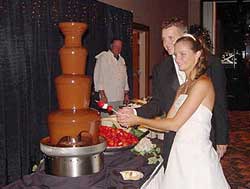In this photograph from a wedding reception, the bride and groom are captured mid-action as they prepare to dip skewers with strawberries and marshmallows into a large four-tier chocolate fountain. The fountain, with its silver base, is prominently placed on a table adorned with a black tablecloth and a white front, accompanied by a large bowl of strawberries. The bride, dressed in an elegant white wedding gown and a matching hair band, stands in the foreground with her long brown hair cascading over her shoulders. She is smiling blissfully as she holds the skewer, while the groom, clad in a classic black tuxedo with a white shirt, stands closely behind her, his hand over hers, sharing in the joyful moment. Behind the table, a chef in a white button-up jacket and gray pants supervises the scene, all set against the backdrop of a black curtain that partially conceals a doorway with a blue frame. The rich, brownish-red carpet underfoot adds to the warm atmosphere of the celebration.